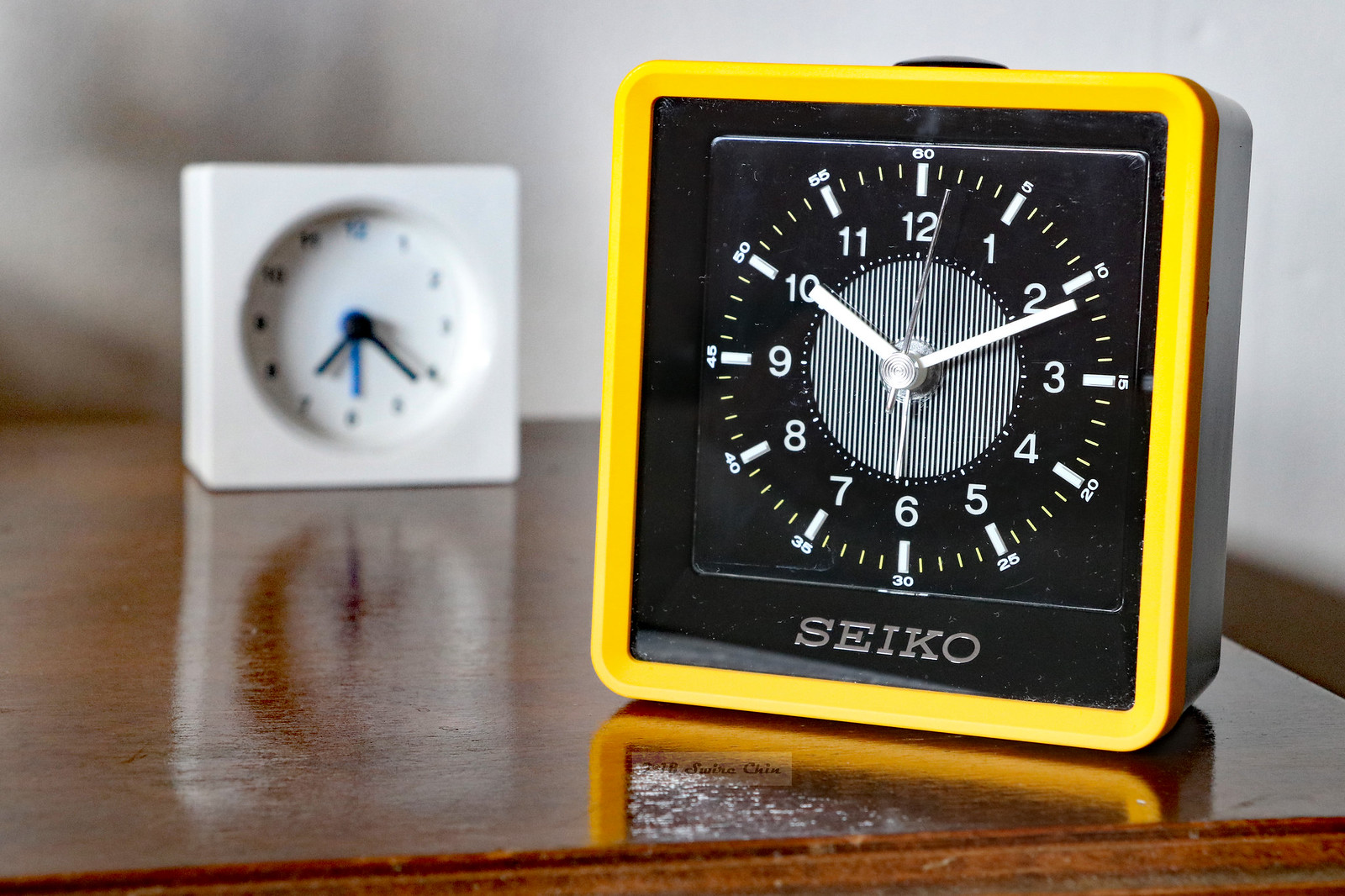A black and yellow square clock labeled "Seiko" is prominently displayed on a shiny brown wooden table. The clock's reflection shimmers on the polished surface. Positioned toward the back of the table is a plain, white square clock, which also casts a mirrored image on the table. In the background, there's a white wall to the right, and on the left side, there are brown horizontal and vertical lines adding an interesting architectural element. The Seiko clock, sitting near the edge of the table, features a noticeable black button on its top.